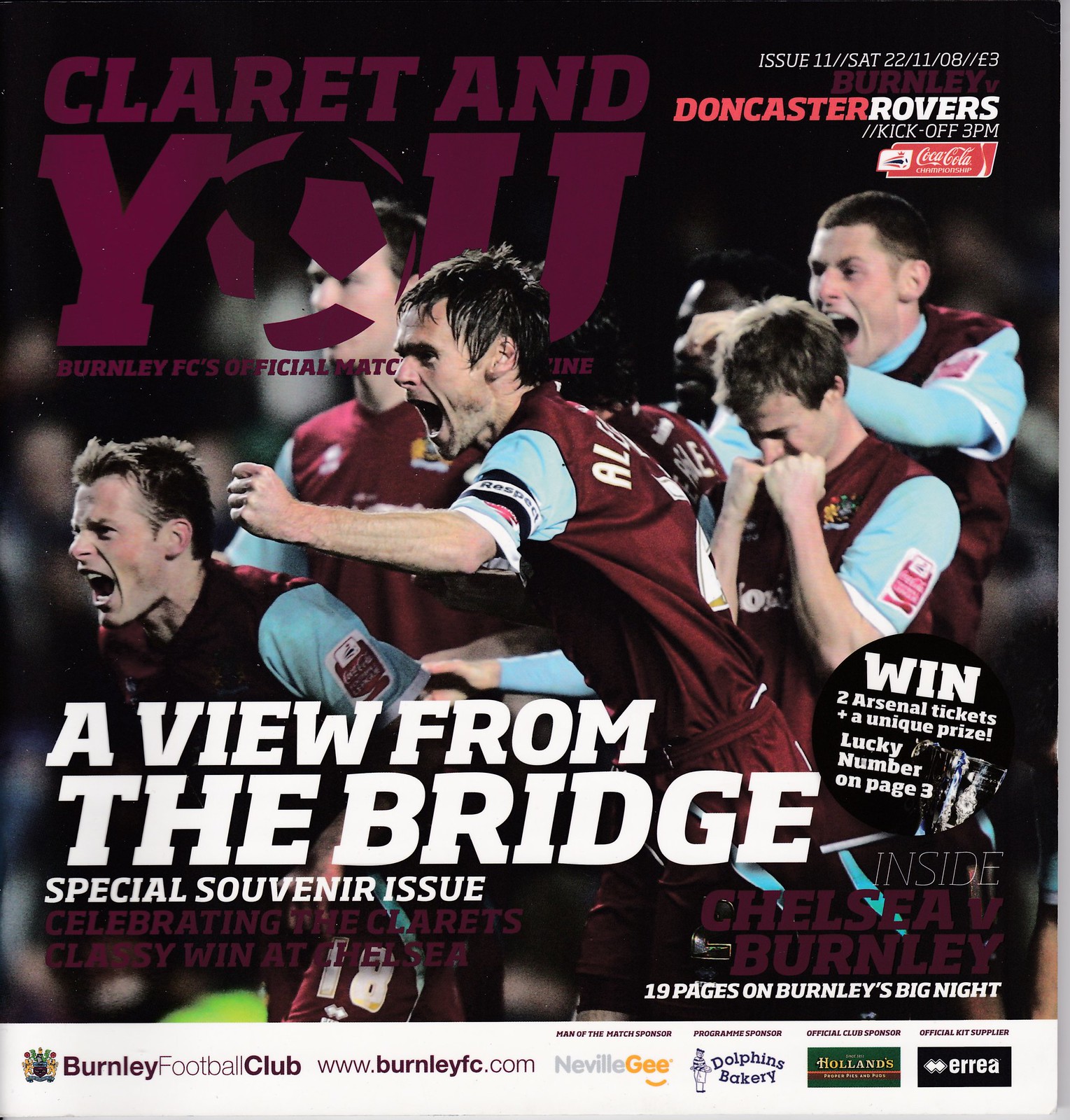The cover of the magazine, titled "Claret and You: Burnley FC's Official Match Day Magazine," features Issue 11 dated Saturday, November 22, priced at £3. The issue details the match between Burnley and Doncaster Rovers, which kicks off at 3 p.m. The cover is dominated by an image of Burnley FC players in burgundy and teal jerseys, celebrating on the field with cheers and raised arms. Bold white lettering announces "A View from the Bridge," highlighting a special souvenir edition celebrating Burnley's classy win against Chelsea. Additional features include a chance to win two Arsenal tickets, a unique prize with a lucky number on page 3, and 19 pages covering Burnley's big night. The overall design features colors such as gray, purple, green, red, tan, and yellow, typical of what you'd find in an official football program handed out at a soccer arena.